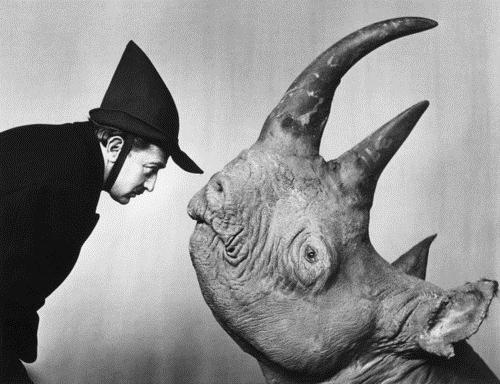In this striking black-and-white photograph, a Caucasian man and a rhinoceros are captured in an intense, almost intimate moment. The rhinoceros, positioned at the bottom right of the image, gazes upward with its head lifted, showcasing its two horns—an elongated, curved one closer to its mouth, and a shorter, straight one behind it. Its ears are tucked back, eyes open, and mouth closed, presenting a still and serene demeanor. On the left, the man, dressed in a black jacket and a distinctive pointed hat with a brim that nearly touches the rhino's nose, leans slightly towards the animal. His hat, secured under his chin, accentuates the closeness of their encounter. His hands are tucked under his stomach, allowing only his face and upper torso to be visible. The grainy background transitions from a whiter grey at the center to darker shades of grey towards the edges, adding depth and context to the photograph.